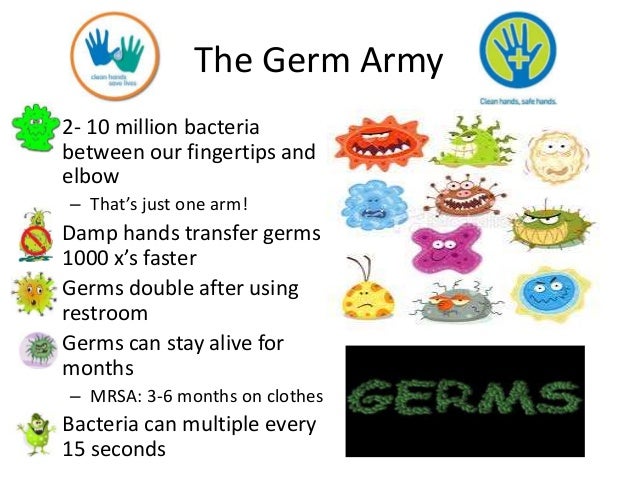This image is an educational poster, likely designed for a doctor's office or a school setting, with a focus on teaching children about germs. The background is white, and at the top in black text, it says "The Germ Army." 

On the left side of the poster, there's a logo featuring two handprints inside a white circle outlined in orange, with the words "Clean hands save lives." On the right side, there's another circle with a green center and a blue hand with a green cross, accompanied by the phrase "Clean hands, safe hands."

The main content of the poster includes several bullet points, each illustrated with cartoon-like germs that have various facial expressions ranging from scared to angry. These bullet points provide information about germs:
- "2-10 million bacteria between our fingertips and elbow. That's just one arm."
- "Damp hands transfer germs 1000 times faster."
- "Germs double after using the restroom."
- "Germs can stay alive for months."
- "MRSA: 3-6 months on clothes."
- "Bacteria can multiply every 15 seconds."

The bullet points are scattered across the poster without a particular center alignment, adding to the cartoony and engaging feel. The colors used in the illustrations and bullet points include blue, green, orange, white, black, yellow, red, and purple. Toward the bottom right corner, there's a black rectangle with the word "germs" written in green, above which are more cartoon depictions of germs.